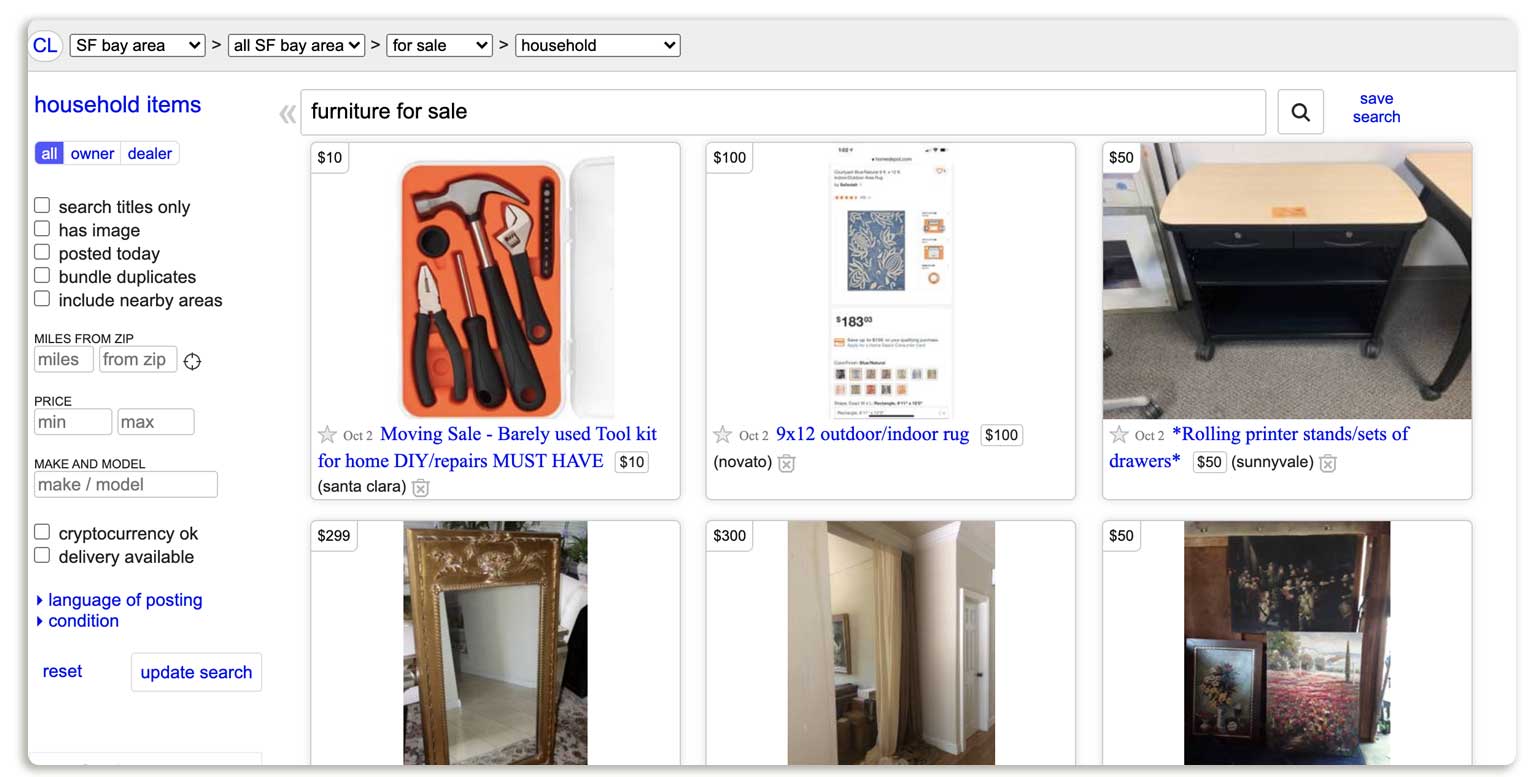A screenshot of a Craigslist search results page for household items, specifically "Furniture for Sale," is displayed. The familiar Craigslist layout is evident, with various category filters on the left that include options like "Search Titles Only," "Has Image," "Posted Today," "Bundle Duplicates," and "Include Nearby Areas." At the top left, just beneath the search bar where "Furniture for Sale" is input, multiple listings are visible within the captured section. The topmost listing is a "Moving Sale: Barely Used Tool Kit for Home DIY Repairs, Must Have," featuring a photo of an orange tool kit containing items such as a hammer and pliers, priced at $10. Following that, a 9x12 Outdoor Indoor Rug is listed at $100. Further down, a Rolling Printer Stand with a set of drawers is available for $50. The lower portion of the screenshot shows listings partially visible, including a mirror priced at $200 on the bottom left.